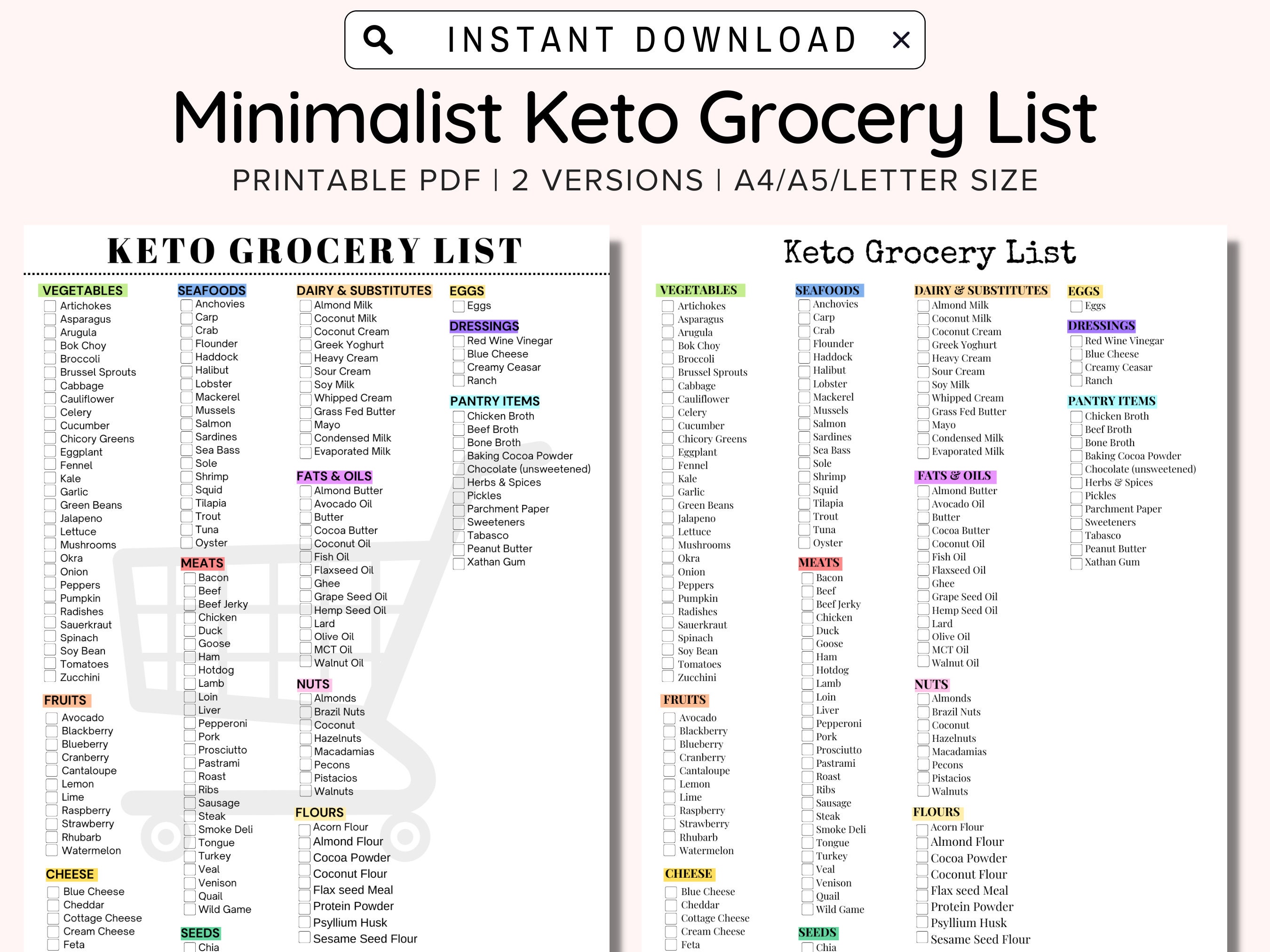This image showcases an advertisement for an instant download of a Minimalist Keto Grocery List in a printable PDF format, available in two versions: letter size. At the top of the ad, encased in a white rounded rectangle with black outlining, the words "Instant Download" are prominently displayed with a magnifying glass icon to the left of "instant" and an "X" to the right of "download." Below, in bold, large print, the title "Minimalist Keto Grocery List" is featured, and further down, it states "Printable PDF" with two available versions. The image depicts two nearly identical grocery lists side-by-side. Each list is organized into categories such as vegetables, fruits, dairy, eggs, cheese, seafood, meats, seeds, substitutions, fats and oils, nuts, flours, dressings, and pantry items, all highlighted in different colors. Each category contains a list of foods with checkboxes for easy shopping. The list on the left has bold headings and a white shopping cart emoji in the background, while the list on the right uses a smaller, less bold font for the headings and lacks the shopping cart design. The emphasis on detail and convenience aims to attract buyers looking for a streamlined, printable keto shopping experience.